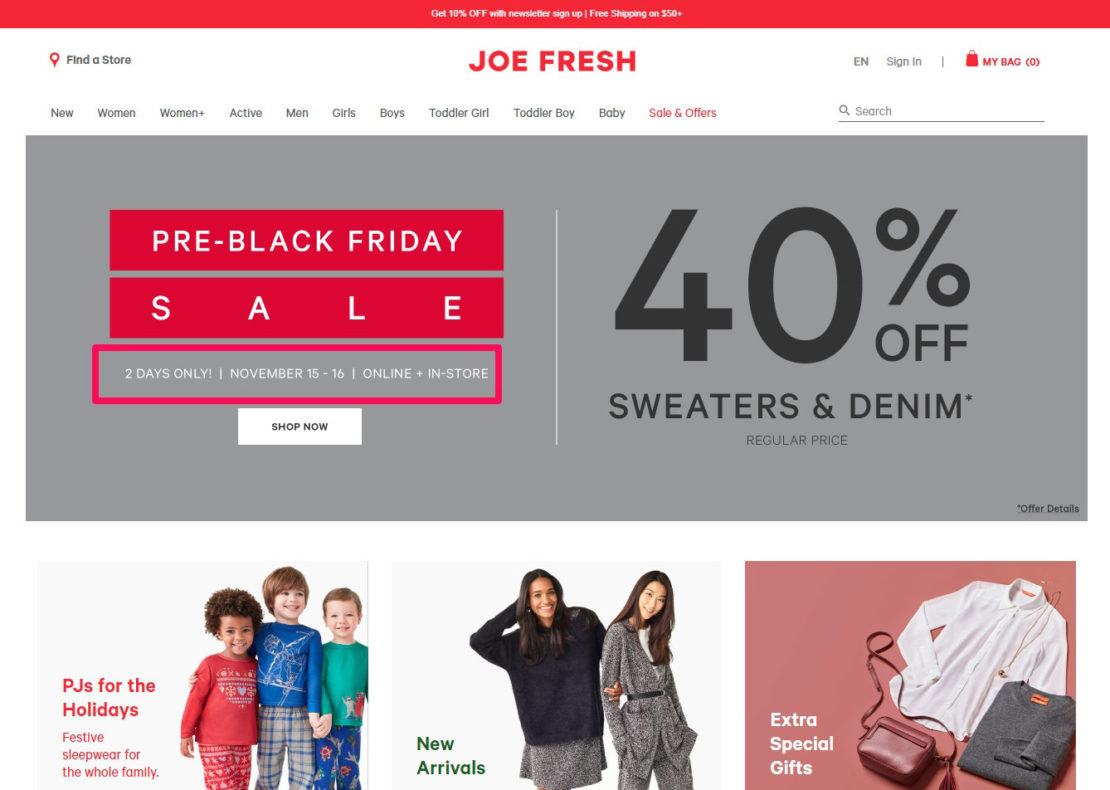The image showcases a promotional webpage for Joe Fresh with various offers and product highlights. 

At the top of the screen, there is a prominent red banner with white text announcing: "Get 10% off with newsletter sign-up, free shipping on $50." Following that, a red header displays "Joe Fresh" on the right, with a "Find a Store" option on the left. Below this, a navigation menu lists categories including: "New Women," "Women Plus," "Active," "Men," "Girls," "Boys," "Toddler Girl," "Toddler Boy," "Baby," and "Sales and Offers," alongside a search menu.

Directly beneath, another red banner states "Pre-Black Friday Sale." Within a white square, emphasized in bold black text, it mentions: "Two days only, November 15th and 16th online and in-store." Below this, in another white box with black text, is the call-to-action button "Shop Now." 

To the right, a highlighted promotion announces, "40% off sweaters and denim (regular price)." Further down, the section labeled "PJ's for the Holiday" features festive sleepwear for the entire family and shows an image of three children, two boys and a girl, wearing pajamas. Adjacent to this, under "New Arrivals," another image shows two girls, with one girl affectionately linking arms with the other. Finally, the "Extra Special Gifts" section displays images of a long sleeve white shirt, a necklace, a gray t-shirt, and a bag, suggesting gift ideas.